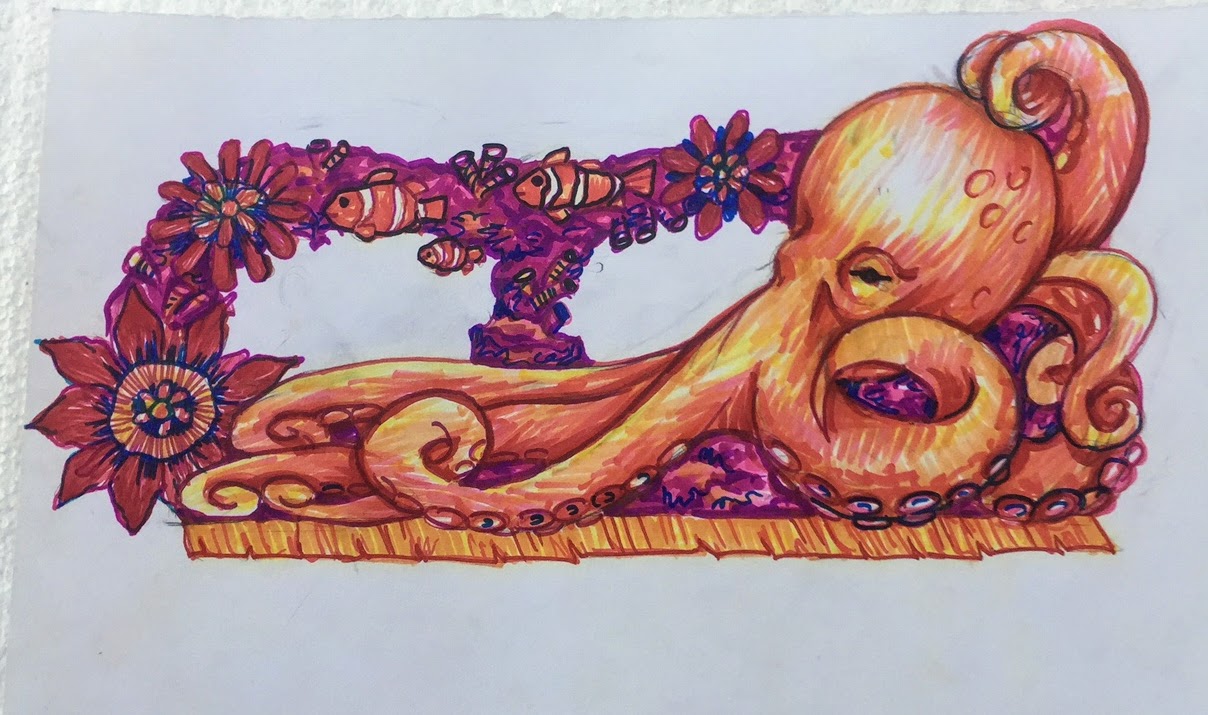A mixed-media artwork, created with pencils and markers, depicts an octopus sprawled on its belly, extending its tentacles forward. Two of its tentacles are curled behind it, resembling a makeshift seat. The octopus is resting on a wooden plank. To its right, a ship's handrail, now overrun by vibrant sea anemones and sea flowers, adds an element of rustic charm. Interestingly, clownfish hover at eye level with the octopus, suggesting a marine environment despite the absence of any visual cues indicating water.